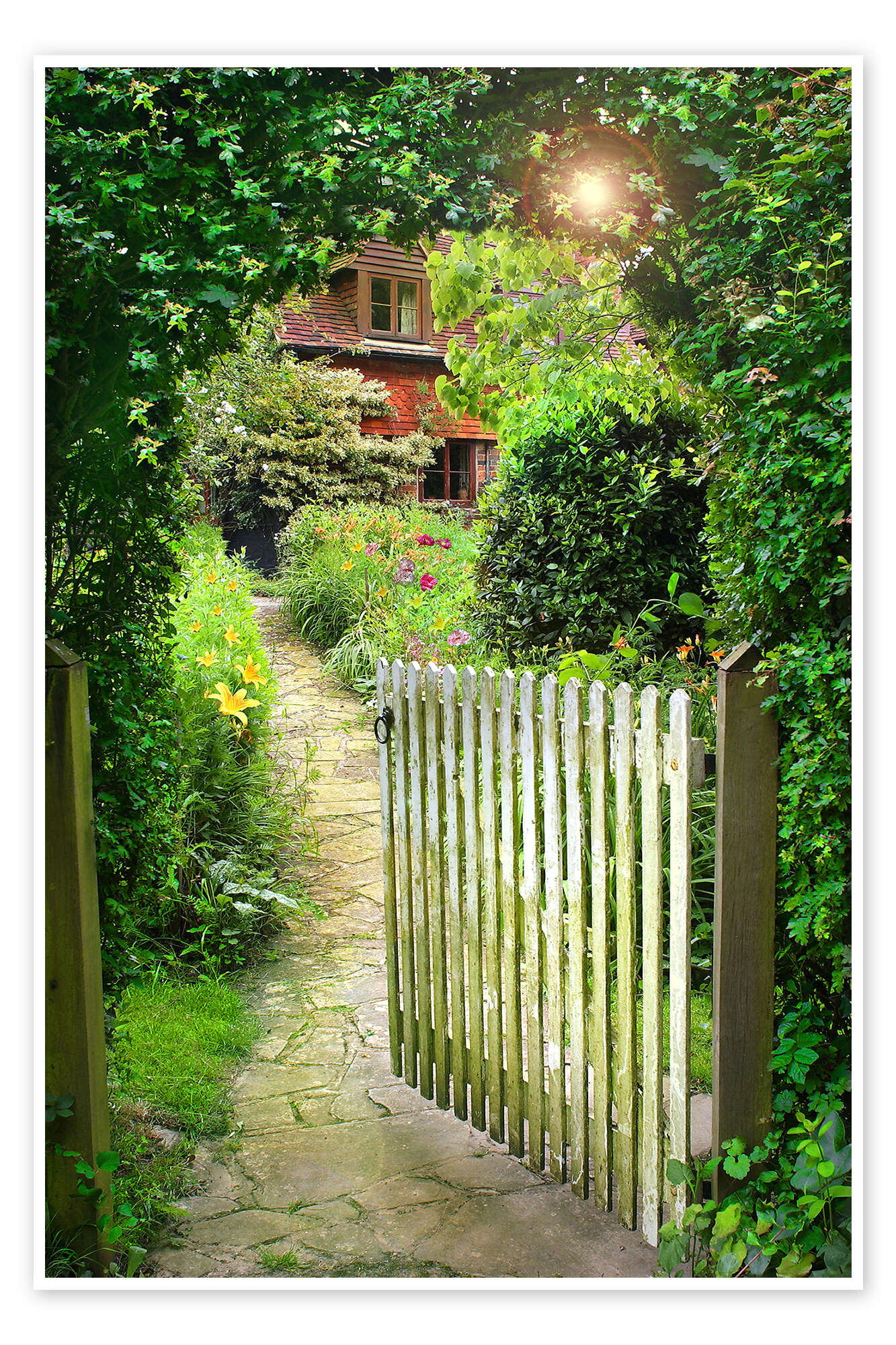This photograph captures a serene garden scene with a prominent brown tiled path leading from the bottom center of the frame toward a distant, characterful house. At the beginning of the path stands a slightly open, white picket gate adorned with splotches of green mildew, hanging between two sturdy wooden posts. A black handle is noticeable on the gate, and the left post has a fastening mechanism attached. The path is flanked by verdant bushes brimming with flowers, predominantly yellow, with some pink and purple blooms on the right. Overhead, a lush archway of green foliage frames the gate, through which the sun peeks, emitting a bright white light and an orange lens flare in the top right corner. The end of the path reveals a visually striking house: the lower level features red brickwork, while the upper level is constructed from brown wood with a mottled red and purple shingled roof. The building has a pair of windows on both the top and bottom levels and is partially obscured on the left by a large, gray bush. The entire scene exudes a secluded, wooded charm, enveloped in abundant green foliage and shrubbery.